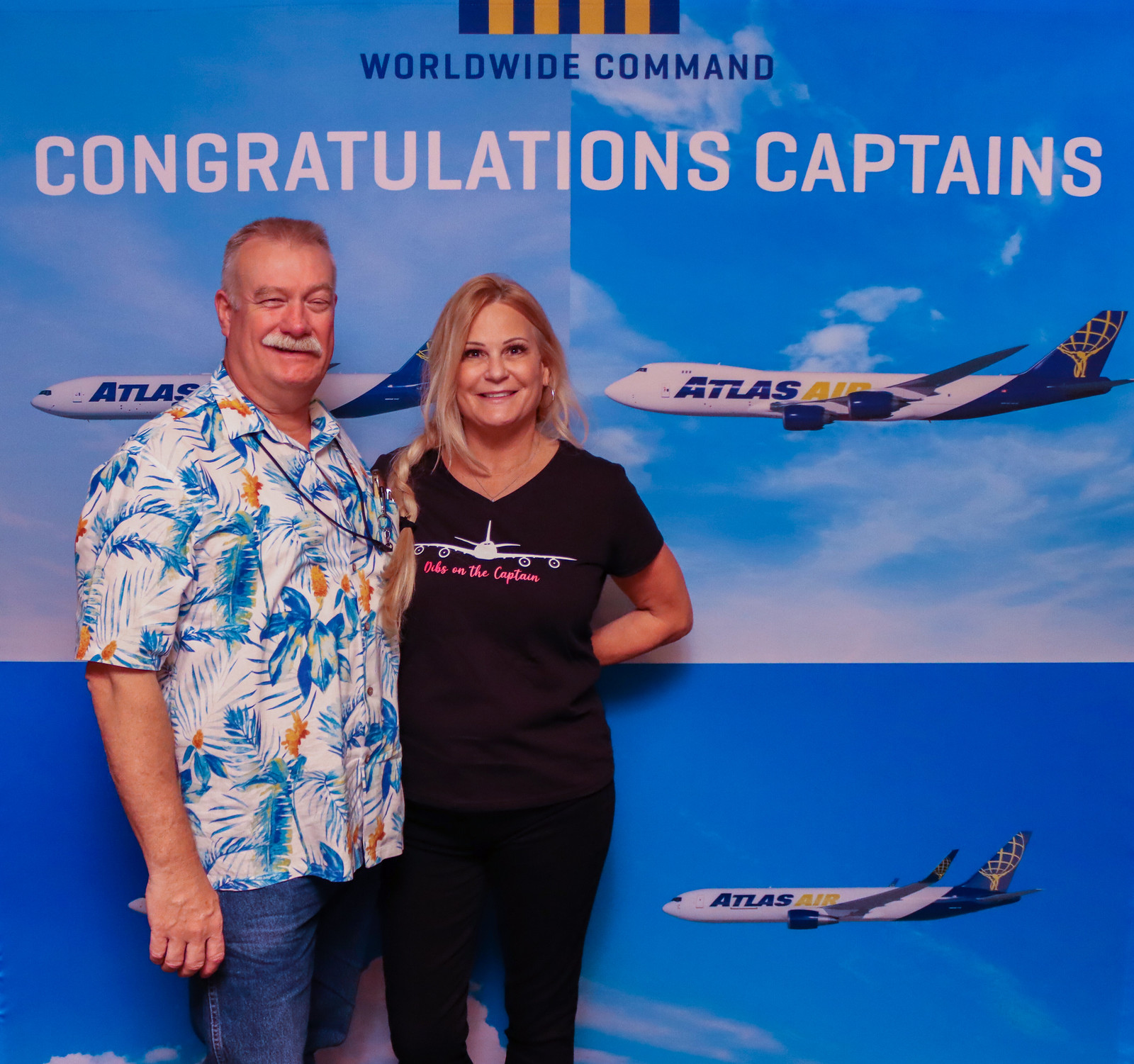In the photo, an older man and a younger woman are standing happily beside each other in front of a vibrant poster that reads, “Worldwide Command - Congratulations Captains!” The poster is a mix of light and dark blue, adorned with three visible pictures of Atlas Air planes soaring through a blue sky. The man, who appears to be in his 50s, sports a graying mustache and short hair that is gray on the sides and brown on top. He is dressed casually in a colorful Hawaiian shirt featuring a blend of blue, white, yellow, and orange foliage motifs, paired with jean shorts. It's a buttoned-up shirt with a collar. Standing to his right, the woman, seemingly in her 40s, has long blonde hair styled in a braid draped over her shoulder. She wears a black V-neck t-shirt emblazoned with an image of an airplane and the phrase “Dibs on the Captain” in pink writing, complemented by black jeans. Both are beaming with joy as they look directly at the camera, their happiness evident in their wide smiles, suggesting a celebratory moment likely connected to their roles as pilots for Atlas Air.